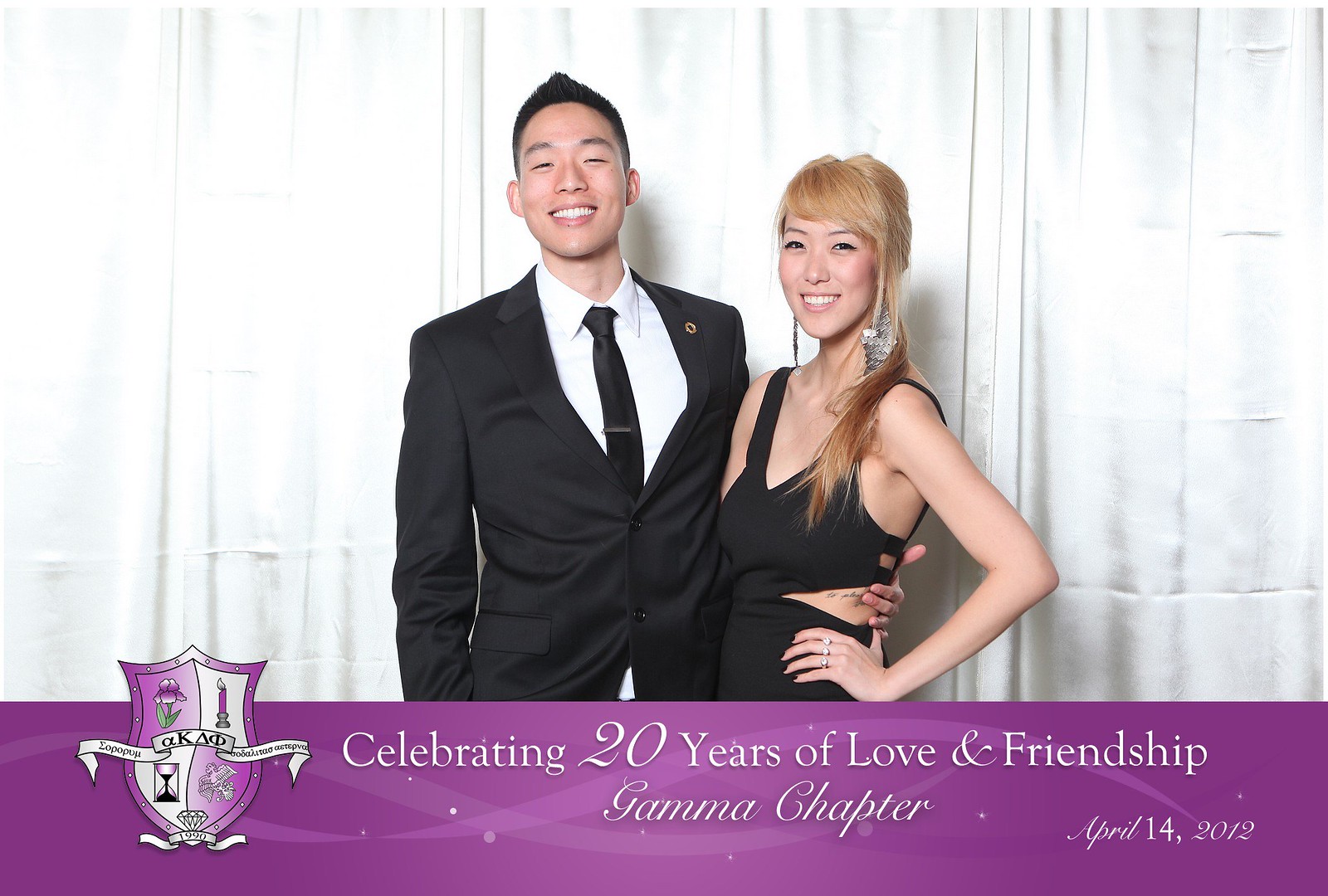This image features a young Asian couple posing against a silver backdrop, celebrating 20 years of love and friendship related to the Gamma Chapter, as noted at the bottom of the photo in purple and white text. The man, taller and with dark hair, is dressed in a dark silky suit with a black tie and a white shirt. The woman, with strawberry blonde hair, wears a black dress adorned with long earrings and three rings on her hand. Both are smiling warmly, capturing the joyful essence of the occasion. The date, April 14, 2012, along with the Gamma Chapter's Greek lettering, further commemorates the couple's longstanding connection, likely stemming from their involvement in the fraternity society they met through.